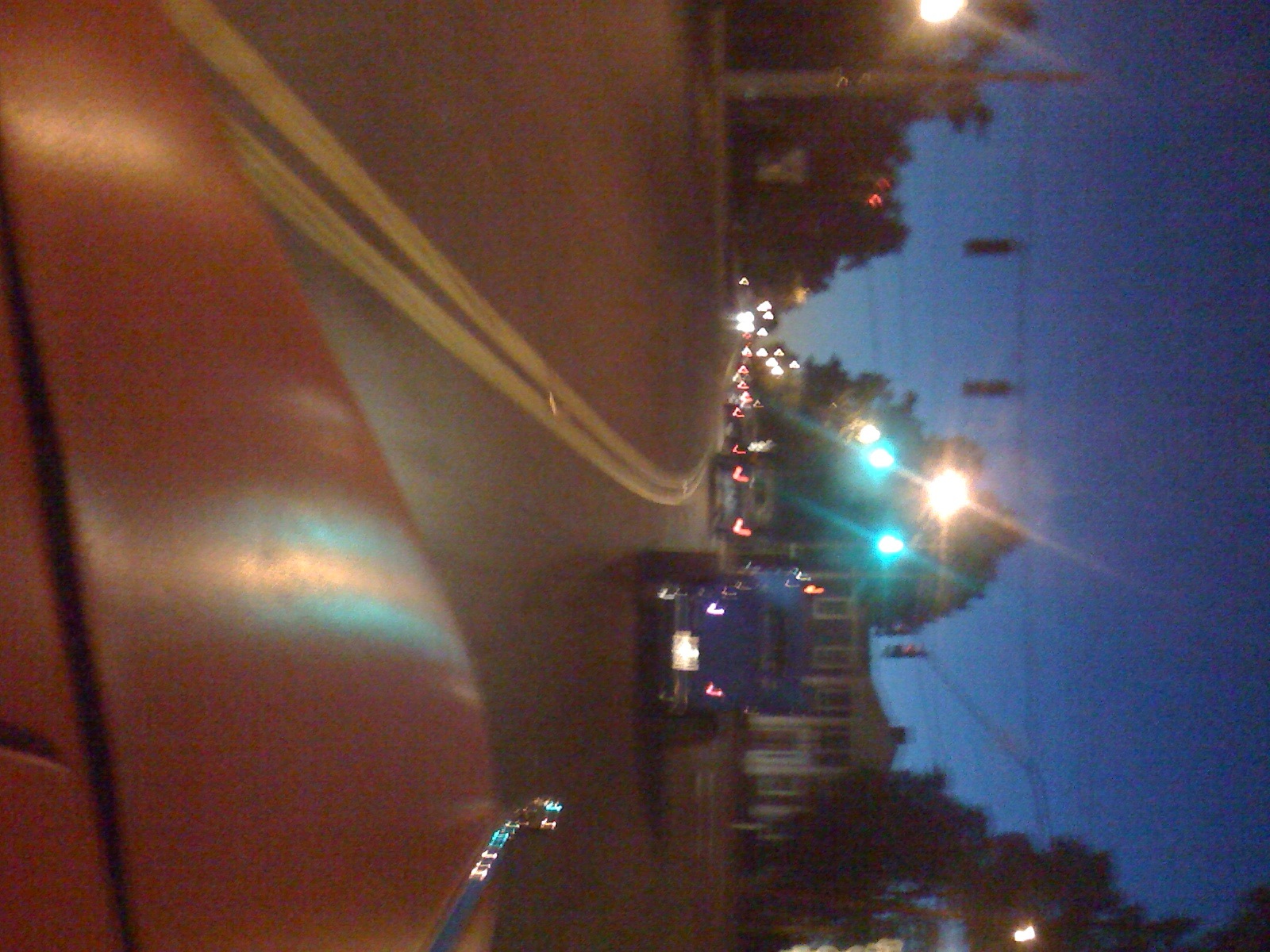This color photo, taken at night from the driver's side of a vintage car, showcases a unique scene on a two-lane road viewed horizontally instead of the intended vertical orientation. The vintage car, distinguished by its red hood and wide rear tires, appears to be made of metal with a carriage-like design. In front of it, a blue car with a rectangular back window can be seen, and further ahead, a third gray car. The street is lined with trees on both sides, and a white house is visible to the right. Several green and strung street lights illuminate the scene, and the sky, despite the darkness, has a distinct blue hue. There is a clear double yellow line marking the center of the road, suggesting one lane for northbound and one for southbound traffic. The image captures the stillness on the opposite side of the road, where no cars are moving, likely halted by a distant traffic light.